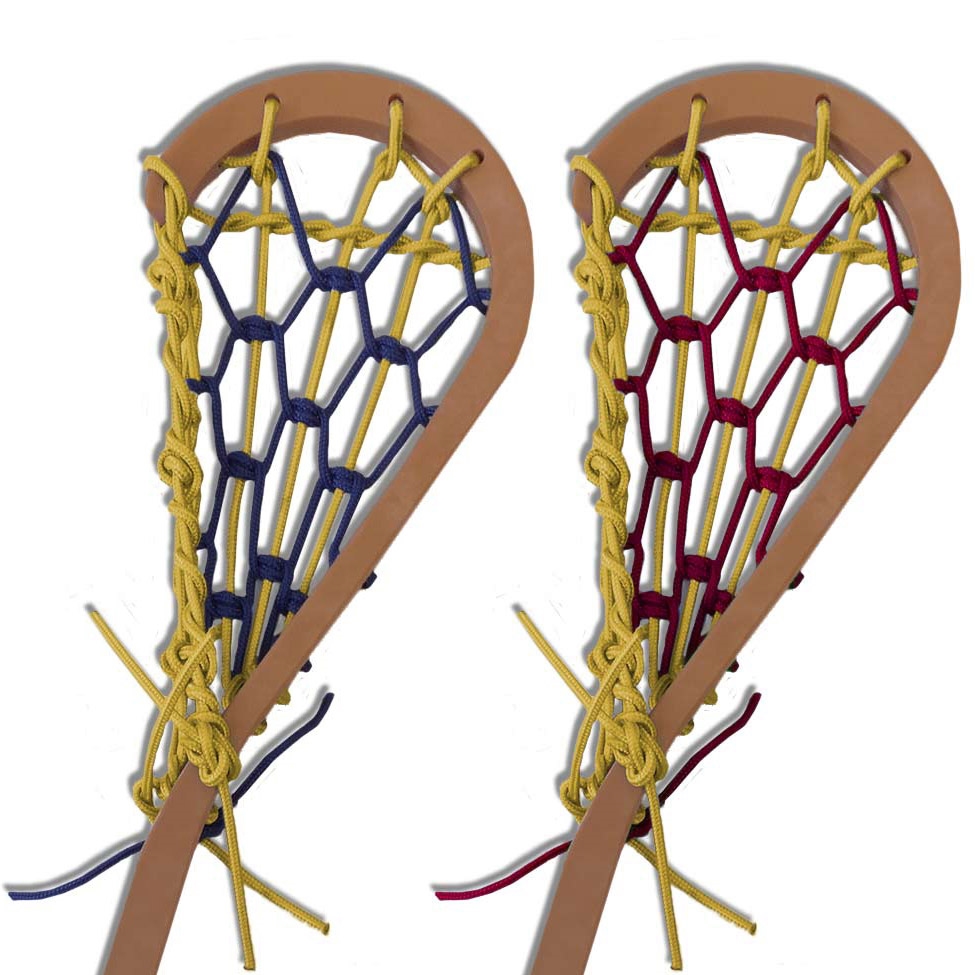The image showcases two intricately designed lacrosse sticks, crafted from brown wood that gently curves into a shape reminiscent of a question mark. Both sticks feature heads that flare out towards the end, forming netted pockets used for catching and throwing the ball. Each stick is adorned with tightly woven leather bindings that secure the netting to the wooden frame, ensuring durability for the sport's demands. The stick on the right has a vibrant red netting in its center, complemented by yellow ropes weaving the top and bottom parts together. Similarly, the stick on the left mirrors this design but with blue netting, maintaining the same yellow rope detailing. Both lacrosse sticks are placed side by side against a stark white, empty background, devoid of any text or additional context.